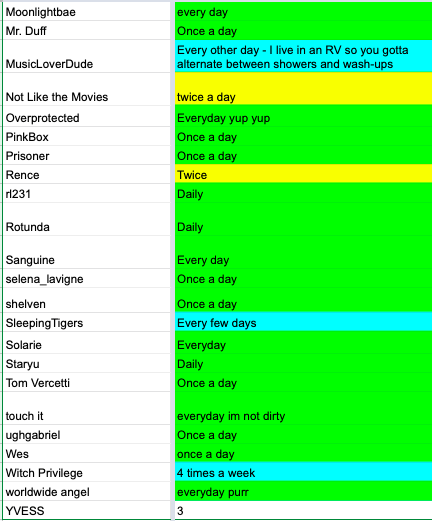A detailed photograph features a rectangular chart, approximately 4 inches tall and 3 inches wide, divided into two halves: a left side with a white background and a right side with neon-colored backgrounds ranging from green to blue to yellow. The chart is bordered by a light green line on the left and bottom edges, with a thin gray border separating the two columns but no border on the right.

On the left side, against the white backdrop with black print, the following names are listed vertically: Moonlight Bay, Mr. Duff, Music Lover Dude, Not Like the Movies, Overprotected, Pink Box, Prisoner, Rents, RT-231, Rotunda, Sanguine, Selena Levine, Shelvin, Sleeping Tigers, Solari, Star U, Tom Brussetti, Touch It, Gabriel, West, Witch Privilege, Worldwide Angel, and U.S.

Corresponding to each name on the right side, the chart displays various frequencies of activities against colorful backgrounds: 
- Moonlight Bay: Green, Every Day
- Mr. Duff: Green, Once a Day
- Music Lover Dude: Blue, Every Other Day ("I live in an RV, so you gotta alternate between showers and wash shops")
- Not Like the Movies: Yellow, Twice a Day
- Overprotected: Green, Every Day ("Yup Yup")
- Pink Box: Green, Once a Day
- Prisoner: Green, Once a Day
- Rents: Yellow, Twice
- RT-231: Green, Daily
- Rotunda: Green, Daily
- Sanguine: Green, Every Day
- Selena Levine: Green, Once a Day
- Shelvin: Green, Once a Day
- Sleeping Tigers: Blue, Every Few Days
- Solari: Green, Every Day
- Star U: Green, Daily
- Tom Brussetti: Green, Once a Day
- Touch It: Green, Every Day ("I'm Not Dirty")
- Gabriel: Green, Once a Day
- West: Green, Once a Day
- Witch Privilege: Blue, Four Times a Day
- Worldwide Angel: Green, Every Day ("Per")
- U.S.: White, 3